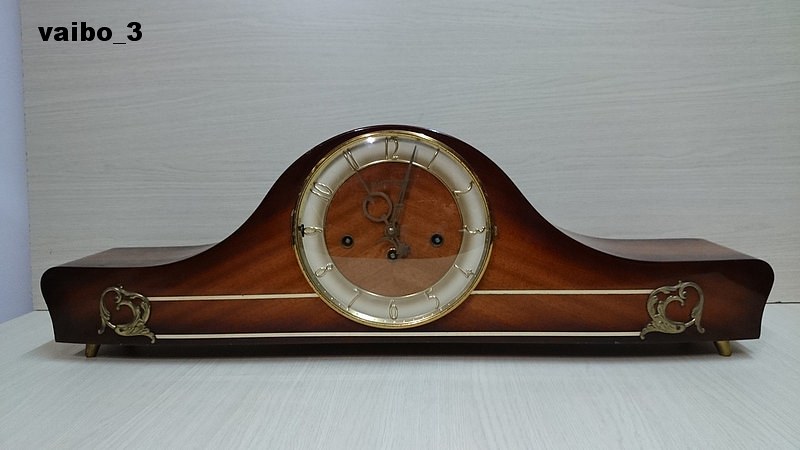This image features a meticulously detailed, vintage Art Deco mantle clock set against a light gray textured background and sitting on a matching gray surface. The upper left-hand corner of the image displays the text "VAIBO_3" in black font. The clock itself is crafted from finely finished wood with a gradient veneer, transitioning from darker edges to a lighter center. The rectangular, yet organically shaped wooden body slopes upward in the middle, resembling a gentle curve akin to an automobile's form, with broader ends tapering towards a larger central section. The clock's face is round and has a pearlized appearance, encircled by a brass ring and showing brass-finished numbers. The hands of the clock, which include a shorter hand distinctive for its circular interruption, are made of bronze. Further adding to its intricate design, the base of the clock is embellished with brass decorations, including lines and leaf-shaped ornaments, resting on small brass feet. The time displayed on the clock reads 11:02.